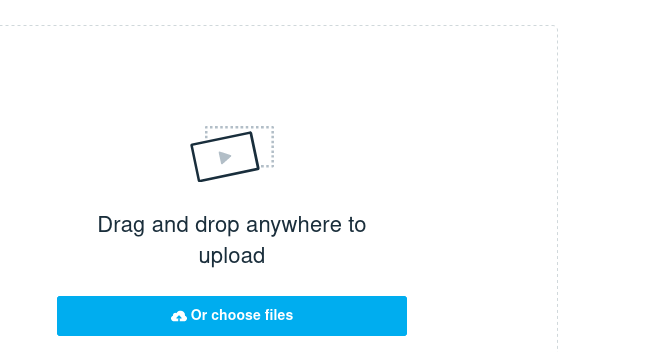The image depicts a user interface for file uploading set against a white background. Central to the design is a small, black-framed rectangle with a white fill, featuring a small gray triangle in its center. Beneath this black-framed rectangle, the directive "Drag and drop anywhere to upload" is clearly displayed in black text. Further down, there is a prominent blue rectangular button. This button is accented with white text that reads "Or choose files," accompanied by a white cloud icon situated to the left of the text. The overall layout suggests a dual functionality: users can either drag and drop files directly into the designated area or click the blue button to manually select files for upload.